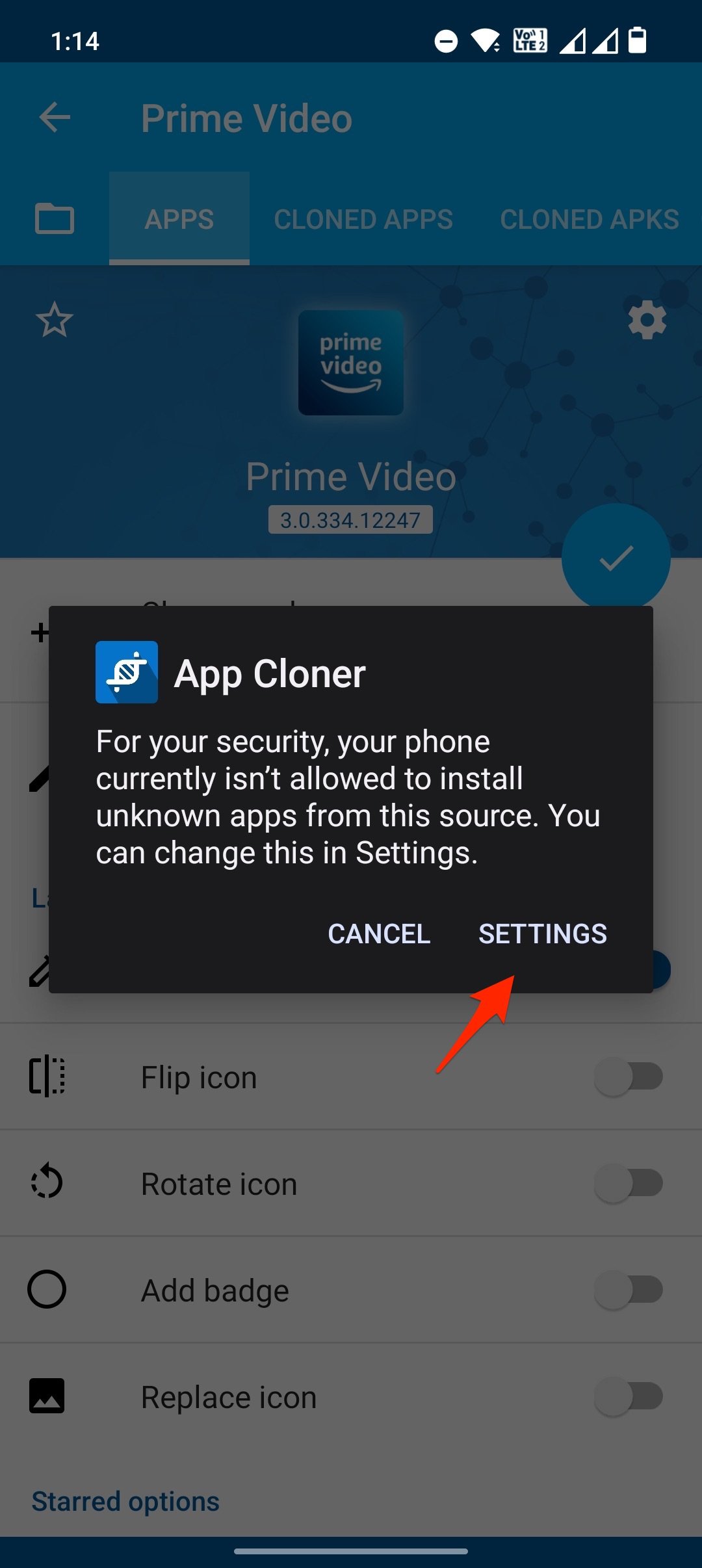The image is a screenshot of a cell phone's screen. At the very top of the screen, the time is displayed as 1:14 PM, accompanied by various status icons. These icons include network connectivity, internet signal strength, and battery level, and they are positioned in the top right corner.

The background of the screen is predominantly black. Faded text near the top of the screen displays "Prime Video," followed by a series of numbers. Towards the right side of the screen, a blue circle with a check mark is prominently visible.

Below this, there is a black rectangle containing text. It reads: "App Cloner," followed by a message warning: "For your security, your phone currently isn’t allowed to install unknown apps from this source. You can change this setting." Below this message, there are two buttons labeled "Cancel" and "Settings." A red arrow points towards the "Settings" button, highlighting it.

Further down the screen, there are options displayed in a lighter, faded color, which include "Flip icon," "Rotate icon," "Add badge," and "Replace icon," each accompanied by corresponding icons. These options are controlled by toggle switches, all of which are currently turned off, as indicated by their gray color instead of blue.

In the bottom left corner of the screen, the phrase "Starred options" appears in blue text.